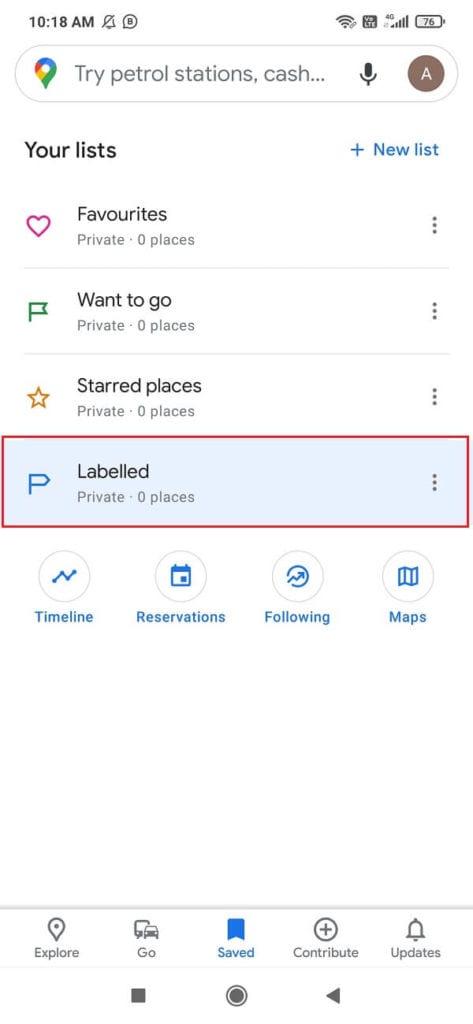This is a detailed screenshot of a cell phone display featuring a Google Maps user interface. The background is predominantly white. 

In the upper left corner, the time is displayed in bold. Adjacent to it on the right, there are two icons. Further to the right, the Wi-Fi, reception bars, battery level, and an additional unidentified icon are visible.

Below this top bar, there's a search bar shaped like a horizontal oval. On the left end of this search bar is the Google Maps icon. The search bar text reads, "Try petrol stations, cash..." in gray font. To the right of this text, there is a microphone icon followed by a brown circle with a white capital "A" inside.

About three lines down, the bolded black text "Your lists" appears on the left side. To the right of this, there is a blue plus sign accompanied by the text "New list."

Directly below this section, a list begins. Each list item has an icon on its left side, followed by a name. The first item is "Favorites," the second is "Want to go," the third is "Starred places," and the last one is "Labeled," which features a light blue background and is outlined with a red border. On the right side of each list item, there's a gray ellipsis for additional options.

At the bottom of the screenshot, there are four circular buttons labeled "Timeline," "Reservations," "Following," and "Maps."